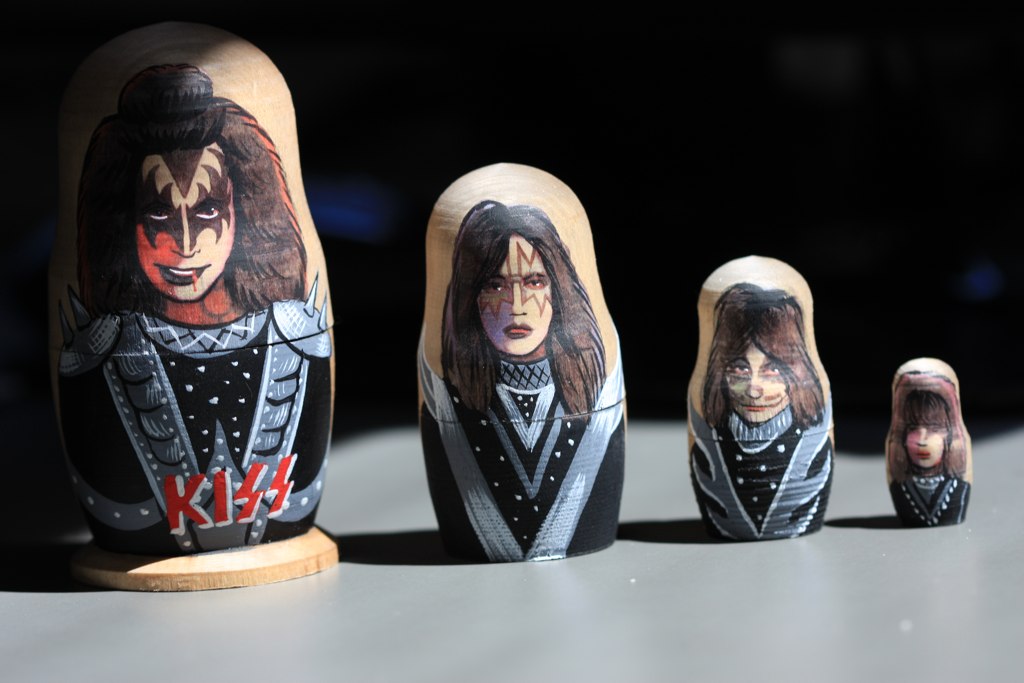This landscape image features a set of four Russian nesting dolls, progressively decreasing in size from left to right, symbolizing band members of KISS. Each doll is expertly carved from wood and painted with distinctive details. The largest doll represents Gene Simmons, easily recognizable by the iconic black and silver face makeup that resembles Batman, along with his elaborate dark outfit and long hair. The word "KISS" is prominently displayed in red, stylized letters at the base of this doll. Subsequent dolls portray other KISS members, each adorned in their characteristic dark clothing and elaborate face paint, maintaining the band's thematic aesthetics. The dolls rest on a pale gray surface, casting shadows to the left, with a black background enhancing the vivid details and colors.